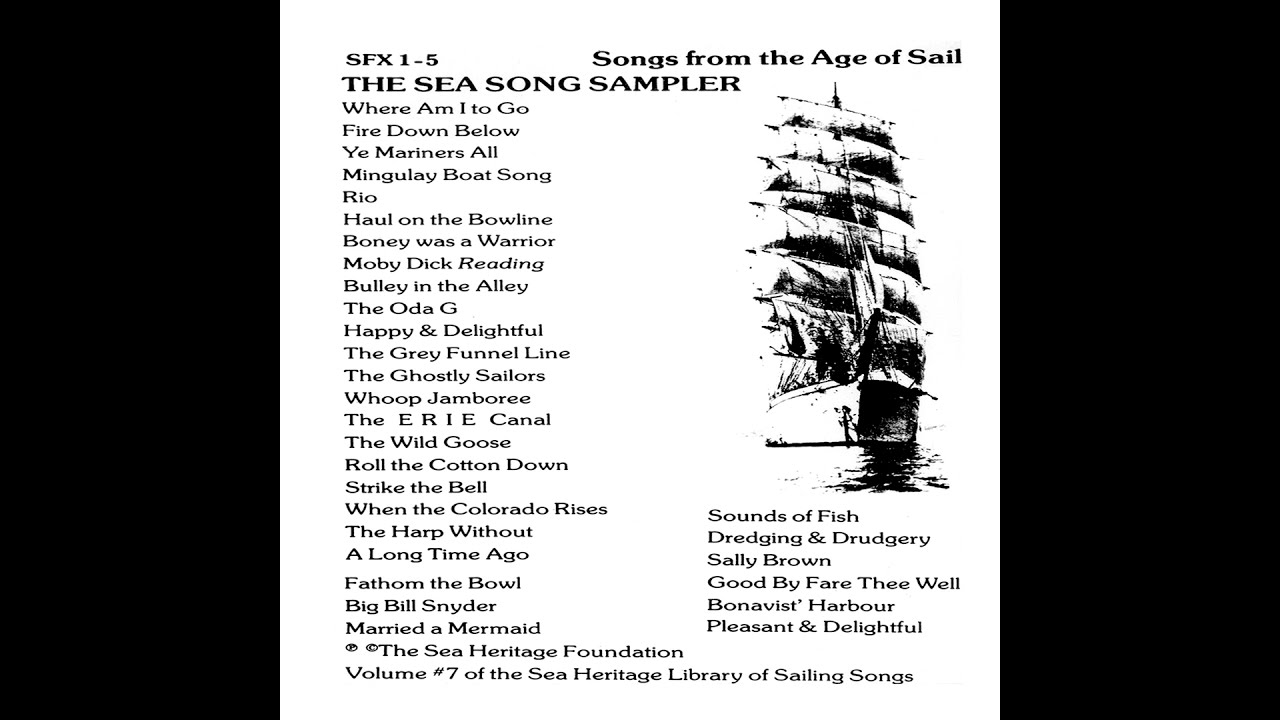This detailed caption encompasses essential details from all three descriptions while emphasizing recurring elements:

The image is a portrait-oriented, black-and-white flyer for an album titled "Songs from the Age of Sail." The top left corner bears the label "SFX 1-5," while the top right corner has the title prominently displayed. Below the title, the subtitle reads "The Seasong Sampler." The main body of the flyer lists songs in black text, including "Where am I to go?" "Fire down below," "Ye mariners all," "Mingoyle Boat Song," "Rio," "Hull on the Bowline," "Boney was a Warrior," "Moby Dick Reading," "Bully in the Alley," "The Ota Gee," "Happy and Delightful," "The Grey Funnel Line," "The Ghostly Sailors," "Whoop Jamboree," "The Eerie Canal," "The Wild Goose," "Roll the Cotton Down," "Strike the Bell," "When the Colorado Rises," "The Harp Without," "A Long Time Ago," "Fathom the Bowl," "Big Bill Snyder," "Married a Mermaid," "Sound of Fish Dredging and Drudgery," "Sally Brown," "Goodbye, Fare Thee Well," "Bonavis Harbor," and "Pleasant and Delightful."

The bottom section of the flyer credits the Sea Heritage Foundation and indicates that this is Volume Number 7 of the Sea Heritage Library of Sailing Songs. To the right of the text, there is a black-and-white faded image of a massive sailboat with several sails, cutting through the water, echoing the seafaring theme of the album.